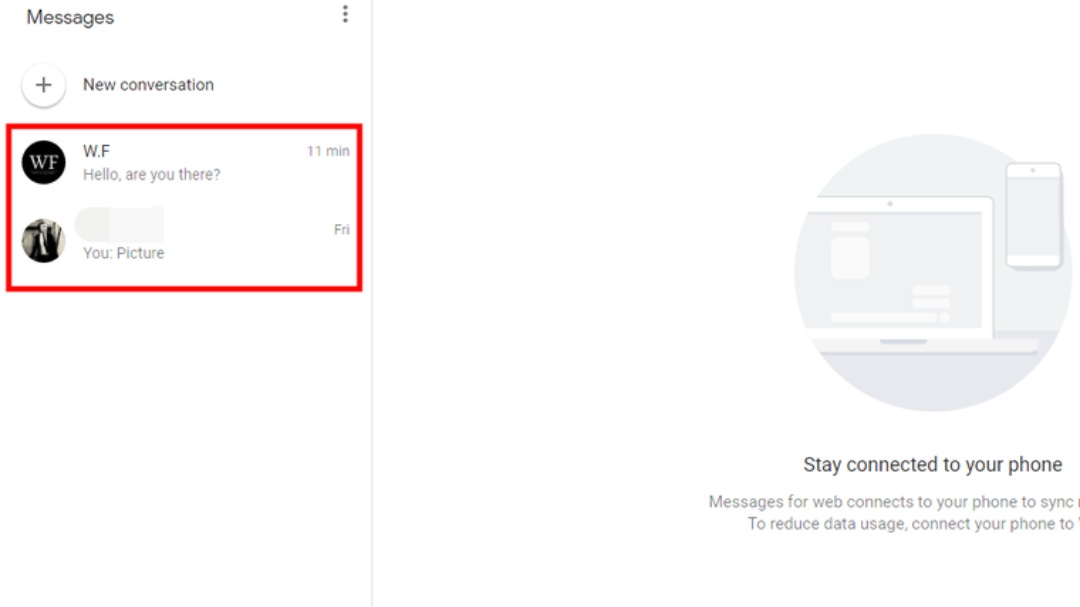A screenshot displaying a desktop or laptop interface, presumably from a "Messages for Web" application, is shown. 

In the image:
1. **Lower Right Text**: There's a block of text in the lower right corner that reads, "Stay connected to your phone. Messages for Web connects to your phone to sync. To reduce data usage, connect to your phone to...".
2. **Vector Graphic**: Above this text, there's a circular vector graphic with a combination of light blue, gray, and white shades.
3. **Main Interface**: The background is predominantly white with a column on the left-hand side. At the top of this column, it says "Messages" next to three vertically stacked dots.
4. **Grey Divider**: A vertical grey divider separates the column from the main screen area.
5. **New Conversation Button**: Below "Messages," there's a button with a plus sign encircled in white listed alongside the text "New conversation."
6. **Red Rectangle Section**: Below this button, a red rectangle is visible. Inside this section:
    - **Avatars**: Two circles, presumably representing user avatars.
    - **Message Preview**: The first avatar, labeled "W.F," accompanies a message reading, "Hello, how are you there?" marked with the timestamp "11 MIN" (likely indicating 11 minutes ago).
    - **Blurred Content**: Below this message, another avatar with a blurred-out name displays "U:" adjacent to a space for an image or text, with "FRI" (likely for Friday) placed to its right.

This detailed breakdown provides a comprehensive view of the "Messages for Web" application interface as captured in the screenshot.